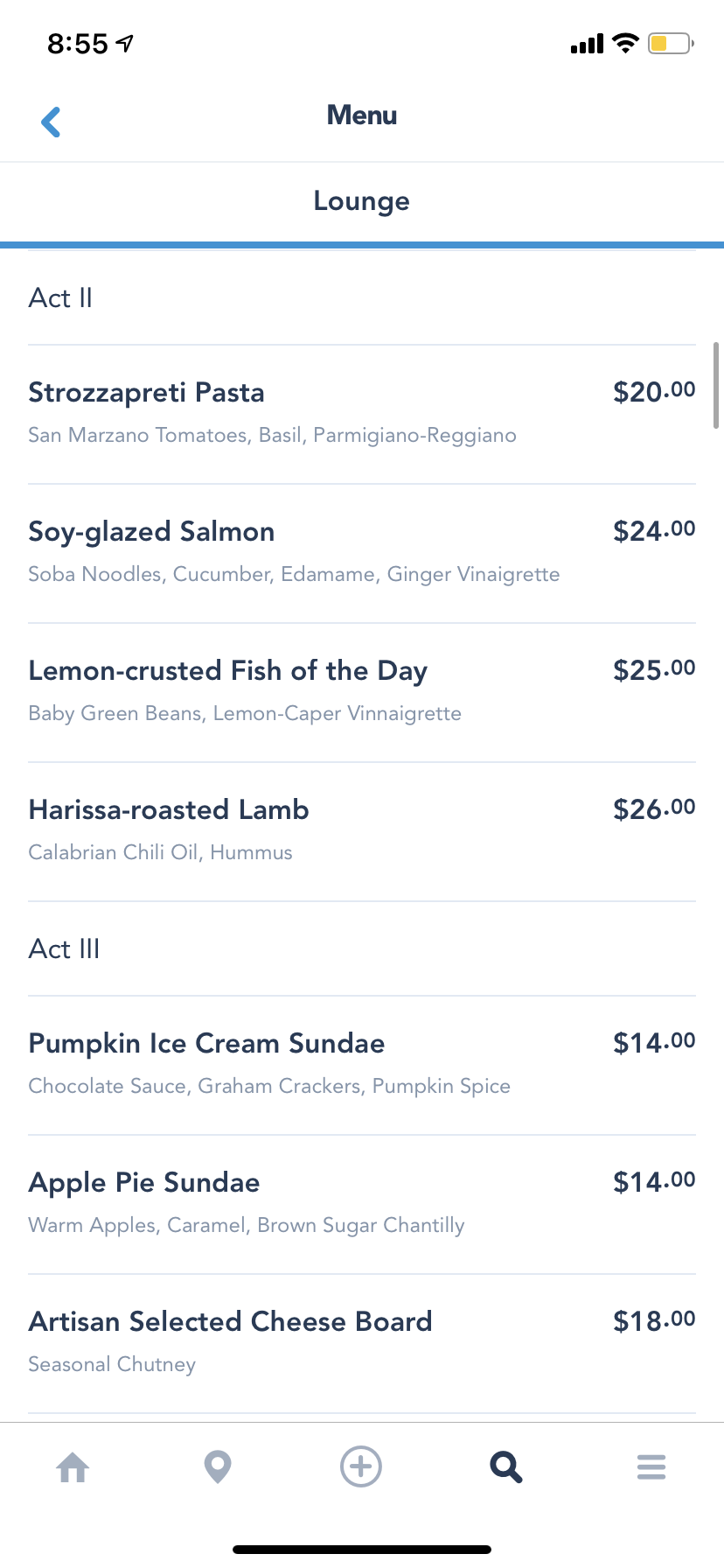On a white background, the screen displays a restaurant menu within an application. In the upper left-hand corner, the time reads 8:55 AM, adjacent to an arrow location icon in black. In the far right corner, various status icons are visible: the cellular signal shows all four bars, the Wi-Fi icon has all three bars filled, and the battery icon is yellow, indicating low power mode with approximately a third of the battery remaining.

Beneath this status bar, on the far left, there is a blue left-pointing arrow. Central to the screen is the term "Menu" in bold black text, with the word "Lounge" below it, both separated by a blue dividing line.

On the left side of the menu, under the gray heading "Act 2," the first listed item is "Strozzapreti Pasta" in black text. The details, "San Marzano tomatoes, basil, Parmigiano Reggiano," follow in gray text, priced at $20. The second item is "Soy Glazed Salmon," accompanied by "soba noodles, cucumber, edamame, ginger vinaigrette," priced at $24. This is followed by "Lemon Crusted Fish of the Day," with "baby green beans, lemon caper vinaigrette," priced at $25. Next is "Harissa Roasted Lamb," with ingredients "Calabrian chili oil and hummus," priced at $26.

Under the heading "Act 3," the first dessert option listed is "Ice Cream Sundae" with "chocolate sauce, graham crackers, pumpkin spice," priced at $14. The next option is "Apple Pie Sundae" with "warm apples, caramel, brown sugar, chantilly," also priced at $14. Finally, the "Artisan Selected Cheese Board" is offered with "seasonal chutney," priced at $18.

At the bottom of the screen, a series of icons are displayed: a house icon, a location icon, a plus symbol icon, a magnifying glass search icon, and a three horizontal line stack icon. Centered at the bottom of the screen is a short black line.